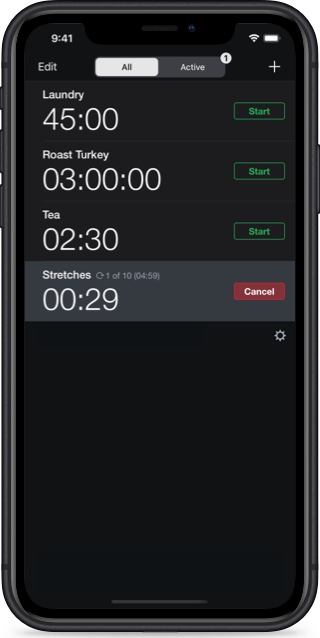The image features a smartphone, presented in a portrait orientation against a white backdrop. The phone, which appears to be a digital rendering rather than a physical device, has a black rectangular frame with rounded edges. On the right side of the frame is a noticeable power button, and on the left side, there are three distinct buttons: two identical ones placed one above the other on the lower part, likely for volume control, and a lone button above them with an unspecified function.

Displayed on the phone's screen is an interface revealing various features and details. At the top, the time reads 9:41, accompanied by a full cell signal indicator and a battery icon with a white meter. Below this status bar is a row with an "Edit" button in white and a toggle switch labeled "ALL" and "ACTIVE." The "ALL" label is highlighted in yellow, indicating it is currently selected, while "ACTIVE" is shown in a gray box with white text.

To the right of this toggle switch is a plus sign, suggesting the option to add more items. The screen lists four tasks, each with specific time durations and associated actions. The first task, "Laundry," is set for 45 minutes and has a rectangular start button featuring a green border, black interior, and the word "Start" in green. The second task is "Roast Turkey" for three hours, accompanied by an identical start button. The third task, "Tea," is scheduled for two minutes and 30 seconds, also with a matching start button. The final task, "Stretches," is set for 29 seconds and instead of a start button, it features a cancel button to the right.

This descriptive caption summarizes the features and interface details of the phone depicted in the image, offering a comprehensive snapshot of its design and functionalities.